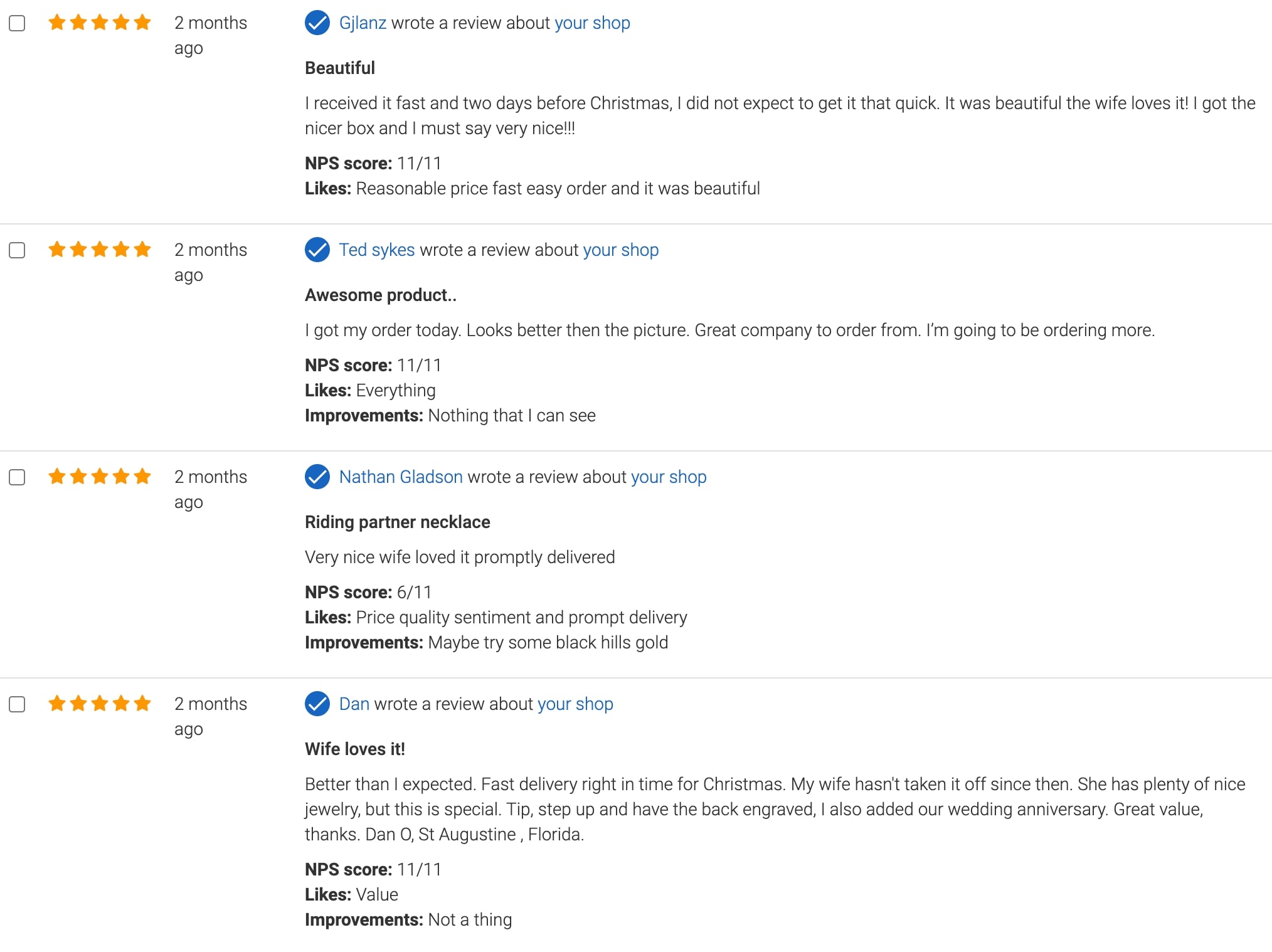The left side of the image features a detailed review section with four rows, each containing an empty checkbox, a five-star rating, and a timestamp indicating "two months ago." Each row includes a customer's review about a shop, their name, and a Net Promoter Score (NPS) out of 11. 

From top to bottom:
1. **Review by G.J. Lenz:**
   - **Review Summary:** Beautiful. I received it fast, two days before Christmas. I did not expect to get it that quick. The wife loves it. It came in a nicer box, and I must say, very nice.
   - **NPS Score:** 11 out of 11
   - **Likes:** Reasonable price, fast and easy order, beautiful product.

2. **Review by Ted Sykes:**
   - **Review Summary:** Awesome product. Got it ordered today. Looks better than the picture. Great company to order from. I'm going to be ordering more.
   - **NPS Score:** 11 out of 11
   - **Likes:** Everything
   - **Improvement:** Nothing that I can see.

3. **Review by Nathan Gladson:**
   - **Review Summary:** Very nice. Wife loves it. Promptly delivered.
   - **NPS Score:** 6 out of 11
   - **Likes:** Price, quality, sentiment, and prompt delivery.
   - **Improvement:** Maybe try incorporating some Black Hills Gold.

Each review offers insights into the customers' satisfaction and provides feedback on what they liked and areas for potential improvement.